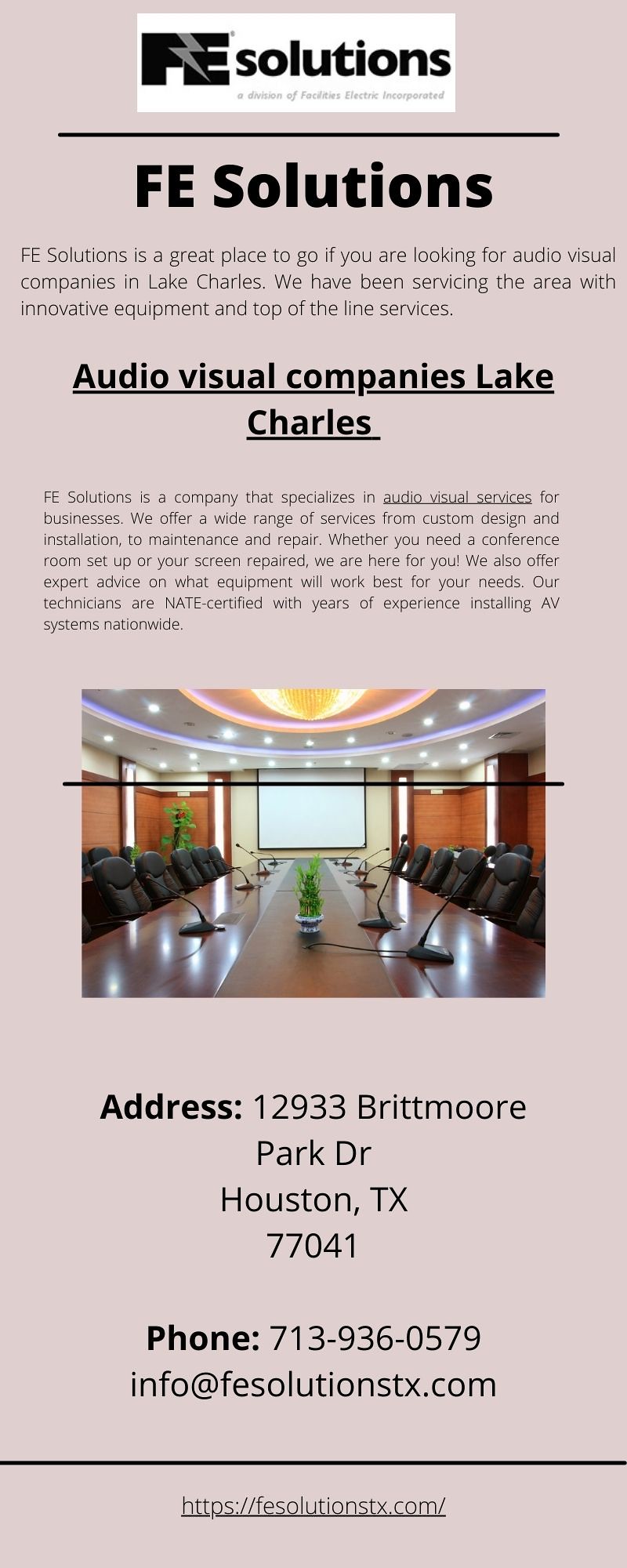The image showcases an advertisement brochure for F.E. Solutions, an audiovisual company servicing Lake Charles. The brochure features a professional boardroom setup centered in the middle, with a dark brown table, black chairs, microphones on both sides, green plants, and a white projection screen positioned behind the table. Above the center image, set against a salmon-colored background with light brown and tan hues on the walls, the text prominently displays "F.E. Solutions" in black, white, and some light accents. The text highlights their specialization in providing top-of-the-line audiovisual services and equipment, mentioning their custom design, installation, maintenance, and repair services. It emphasizes their NAIT-certified technicians with extensive experience in installing A.V. systems nationwide. The contact information, including the address (12933 Brickmore Park Drive, Houston, TX, 77041), phone number (713-936-0579), email (info@fesolutionstx.com), and website (https://FESolutionsTX.com/), is detailed at the bottom. The overall style and setting of the brochure are aimed at promoting F.E. Solutions as a premier choice for audiovisual services in Lake Charles.